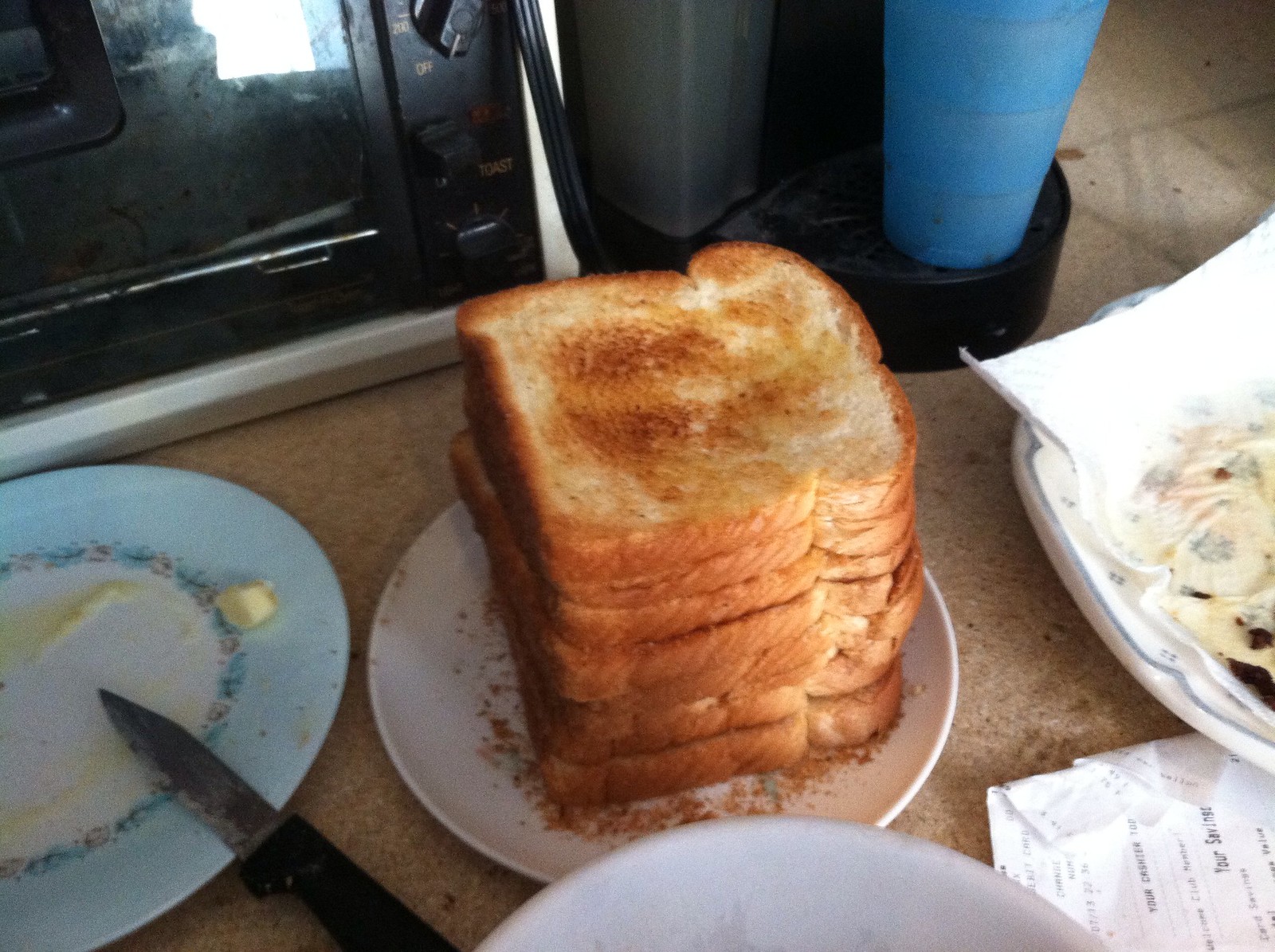In the photograph, a somewhat messy kitchen countertop is depicted. The central focus is a small white dessert plate holding a stack of eight golden-brown slices of toasted white bread, with crumbs scattered around. Adjacent to this plate is another small plate, pastel blue with floral patterns around its white center, which holds remnants of butter and a small paring knife. This suggests the toast was buttered here. A black toaster oven is partially visible in the background, labeled with settings like "toast," and appears quite dirty. There's also a blue cup and a coffee maker nearby. To the right, a plate with a greasy paper towel, possibly used for bacon, further contributes to the overall impression of a cluttered and untidy workspace. A receipt and another white plate with napkins are also visible on the speckled brown countertop.